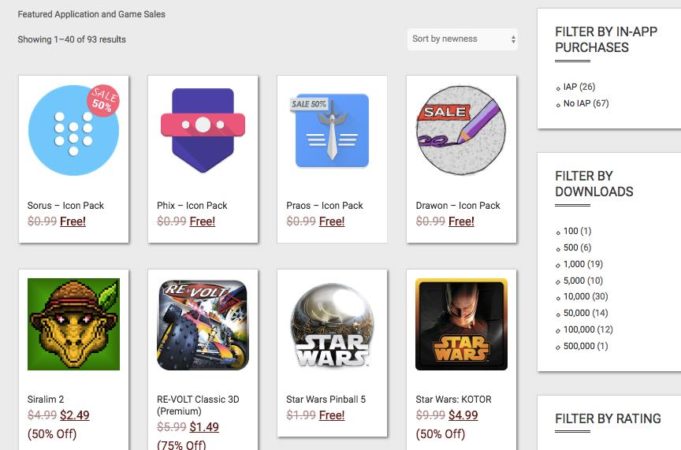The image depicts a screen from an app store, designed for downloading other apps. The background is a light blue color. At the top, black text reads "Featured Application and Game Sales," displaying results 1 to 40 out of 93. On the right side, there's a drop-down menu allowing users to sort the results, currently set to sort by "newness."

The screen is divided into three filter sections: 
1. "**Filter by In-App Purchases (IAP):**" Users can select between apps with in-app purchases (26 results) or without in-app purchases (67 results).
2. "**Filter by Downloads:**" Options include thresholds such as 100, 500, 1,000, 5,000, 10,000, 50,000, 100,000, and 500,000 downloads.
3. "**Filter by Rating:**" This section is partially cut off, making it difficult to read in its entirety.

Below the filter sections, there are app results displayed:
1. **Soros Icon Pack** - Free
2. **Fix Icon Pack** - Free
3. **Preos Icon Pack** - Free
4. **Drawn Icon Pack** - Free
5. **Serial M2** - $2.49
6. **Revolt Classic 3D Premium** - $1.49
7. **Star Wars Pinball 5** - Free
8. **Star Wars: KOTOR** - $4.99